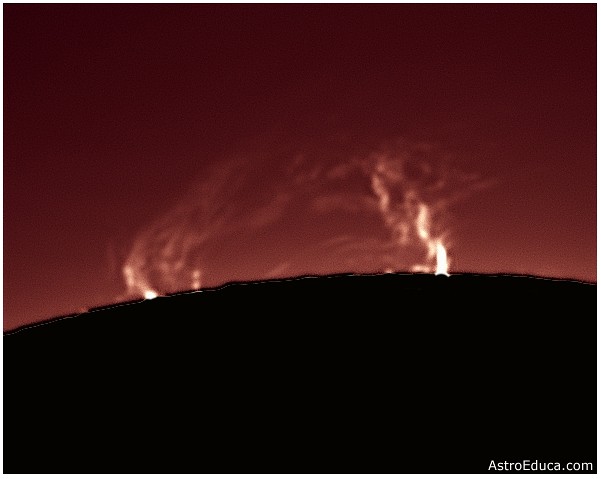This rectangular image, slightly wider than it is tall, captures a dramatic solar scene and is branded with the website address astroeduca.com in the bottom right corner. Dominated by dark tones, the lower half of the image is almost entirely black and forms a curved horizontal line -- likely the edge of the Sun, obscured to highlight solar phenomena. Above this dark curve, a gradient of dusky red and purplish shades, tinged with lighter red near the transition, envelops the upper portion of the image. Strikingly bright, wispy white flames – solar flares – arc upwards from the blackened edge, dissipating into the surrounding reddish, smoky haze. The image's low resolution lends a haunting ambiance to this celestial spectacle.